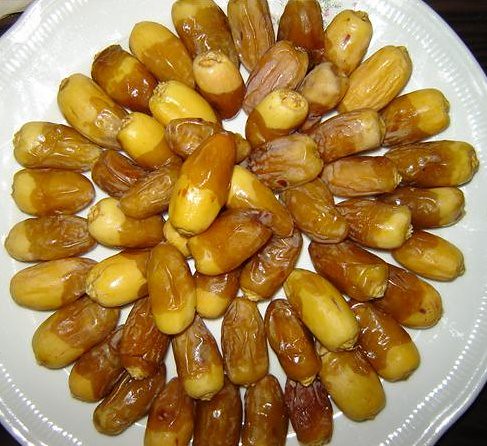The image features a white circular plate adorned with small, horizontal lines around its outer edge, set against a black background that is visible at the corners. On the plate is a tastefully arranged pile of dates, exhibiting a mix of dark brown and light brown hues, with the darker dates mostly at the bottom and the lighter ones near the top. These dates, which appear slightly glazed, are largely arranged in loosely concentric circles around the edge. However, towards the center, they are randomly mounded on top of each other, creating a less orderly appearance. The dates vary in color from light yellow to medium brown, and many display a gradient or spots of dark reddish-brown. Oblong and round in shape, the dates collectively form a visually appealing and somewhat chaotic centerpiece on the elegantly designed plate.